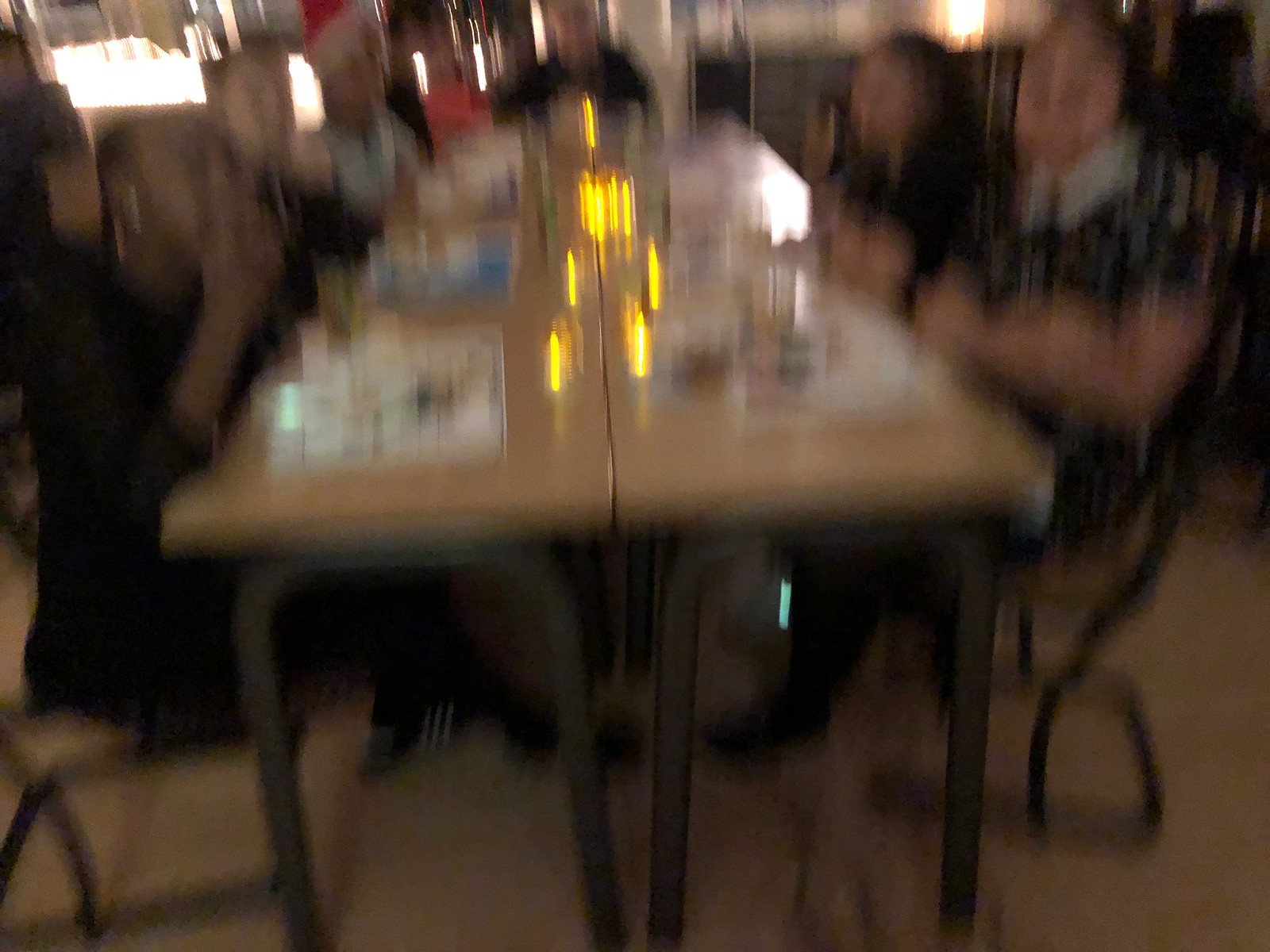This extremely blurry photograph captures a dining scene, likely inside a restaurant. Dominating the center is a long table with a wooden surface and metal-framed legs. Seated on either side of the table are several indistinct figures, appearing as a mix of men and women, many dressed in dark outfits. Notably, one individual towards the back of the table is distinguishable by a red Santa hat. The lighting reflects off water glasses arranged on the table, adding a soft glow to the scene. Additional light sources or possibly reflections are visible along the table’s center, giving the impression of small lights or candles. Despite the blurriness, a person on the front left seems to be eating, raising a hand to their mouth, while another person on the front right wears a flower-patterned dress with a white collar. The overall ambiance hints at a lively dining experience, though the exact details remain obscured by the photo's poor quality.